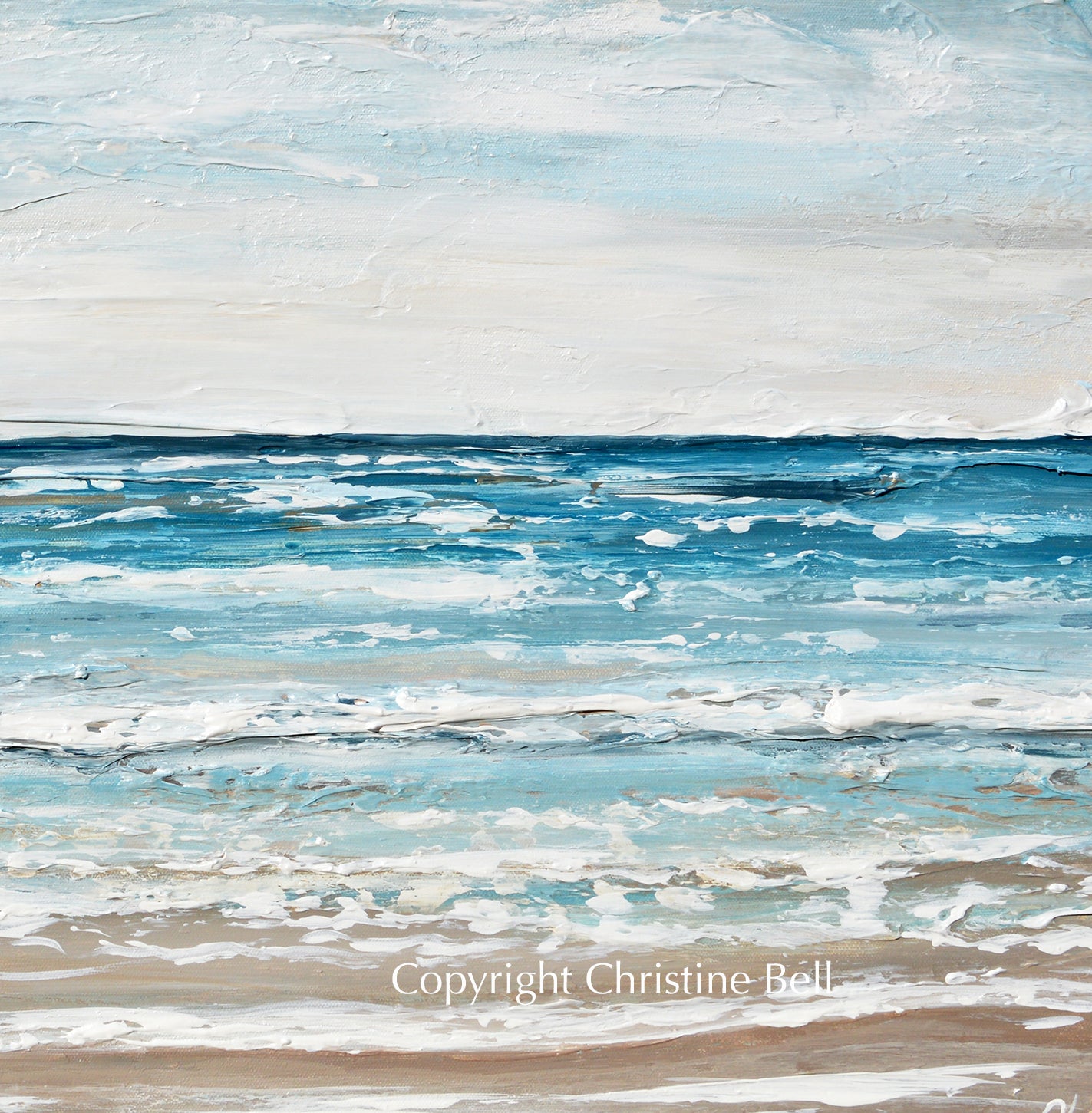This highly textured and detailed painting, titled "Copyright Christine Bell," captures the dynamic beauty of the ocean as it washes up on the shore. The scene begins with dark blue, nearly black waves in the distance that lightens to genuine ocean blue and eventually transitions to a light blue as they move closer to the shore. As the water becomes shallower, shades of gray and grayish blue reveal the sandy bottom, which finally gives way to the gray sand exposed at the very edge. The waves, adorned with white caps, create a vibrant and flowing motion as they crash against the shore, where the sand appears brown mixed with hints of white foam. The sky is pale blue, fading to white near the horizon, with scattered clouds adding a touch of haze. Water droplets leap from the surf, and the overall composition conveys an organic and genuine sense of movement and life. In the bottom right corner of this exquisite portrayal, the artist's signature, "Copyright Christine Bell," is inscribed in white letters.